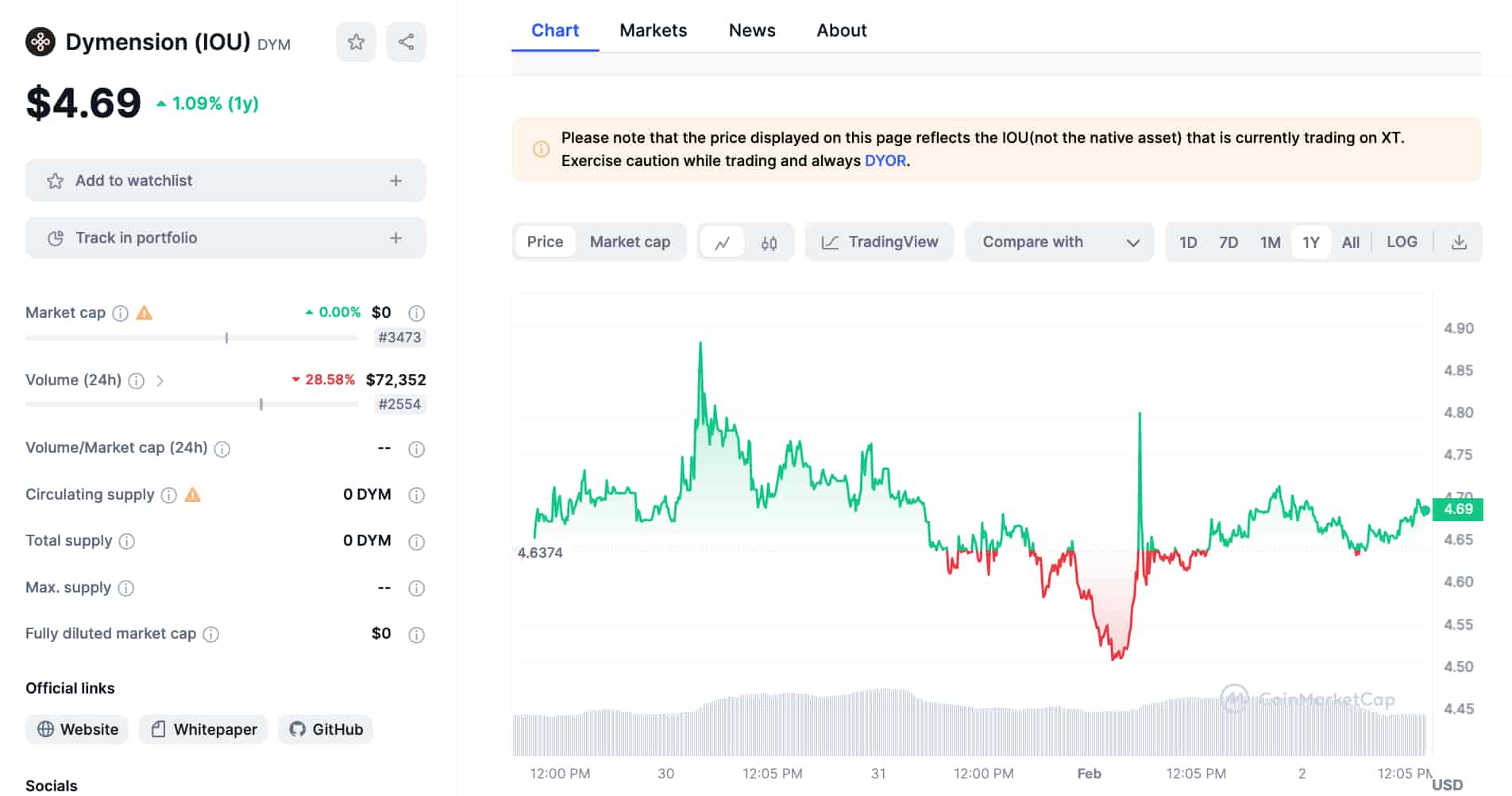This image is a cropped screenshot of the XT trading platform, featuring a sleek interface with a white and black background. In the top left corner, the XT logo is prominently displayed, accompanied by "dimension" in parentheses and black font. Adjacent to the logo, the stock symbol "DYM" appears in small gray letters.

Dominating the left side of the page is a comprehensive information panel. At the top of this panel, the current price per share is shown, indicating a 1.9% increase over the past year. Below this, two gray bars labeled "Add to Watchlist" and "Track in Portfolio" provide quick access to these functions.

Further down the panel, an array of detailed stock information is provided, including Market Cap, Volume, Volume Market Cap, details for the Last 24 Hours, Circulating Supply, Total Supply, Max Supply, and Fully Diluted Market Cap. This section also features "Official Links" with three horizontally arranged boxes linking to the stock's website, whitepaper, and GitHub repository. Notably, the "Socials" section at the bottom left is cropped out of the screenshot.

To the right of the information panel, a large, colorful line graph occupies significant space, with green representing periods of upward performance and red indicating declines. Above this graph, a red alert box with an eye icon stands out, delivering an important notification.

Centrally positioned at the top of the page, there are four category tabs: Chart, Markets, News, and About, with Chart currently selected.